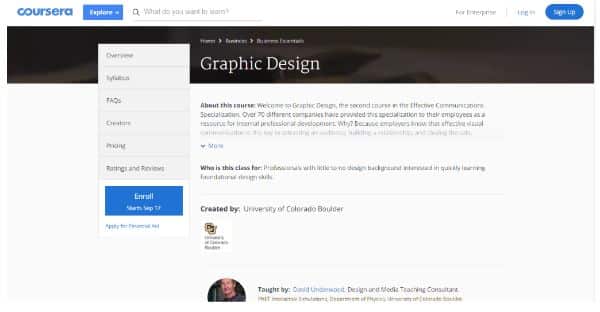A screenshot featuring a light gray background displays the Coursera homepage. Prominently at the top, the "COUR-SERA" logo sits alongside a blue button labeled "Explore." A search bar occupies the center, while on the right side, there are options for "Log In" and a blue oval button labeled "Sign Up."

Beneath the main navigation, the screenshot highlights a course related to graphic design. The section is segmented into various rectangles containing different pieces of information, including an email input field at the bottom.

Detailed descriptions about the course are provided under headers such as "About this Course," followed by a snippet of information and a "More" link in blue. There's also a section titled "Who is this Class For?" which elaborates on the target audience with additional details.

The course is created by the University of Colorado Boulder, featuring a profile picture of a man indicating the instructor. Next to the picture, it says "Taught by" with the instructor's name highlighted in blue. The text in this section is relatively small, providing further information about the course and the instructor.